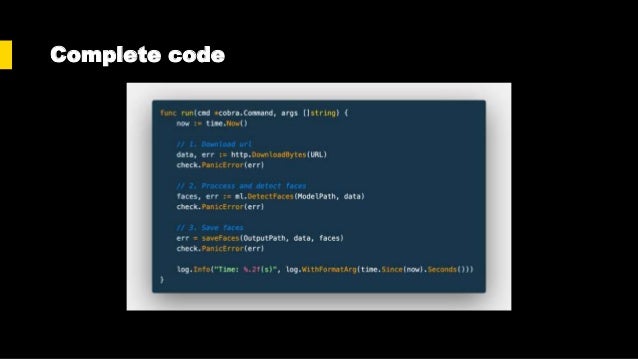This image is a detailed screenshot with a very black border encompassing roughly one third of the image. Near the top left corner, set about a tab space away from the border, is a small yellow rectangle, and next to it in bold white text, it reads "Complete Code." Below this, at the center of the image, there's a picture within a white field that creates a border, which contains a blue-tinted box of code. The code itself is diverse, featuring primarily white, orange, and blue text, with small accents of green and purple near the bottom. The code displayed starts with the line “func run(cmd *cobra.Command, args []string) { now := time.Now()” and continues in a structured format that fills the blue background, providing a detailed and colorful representation of a programming script.